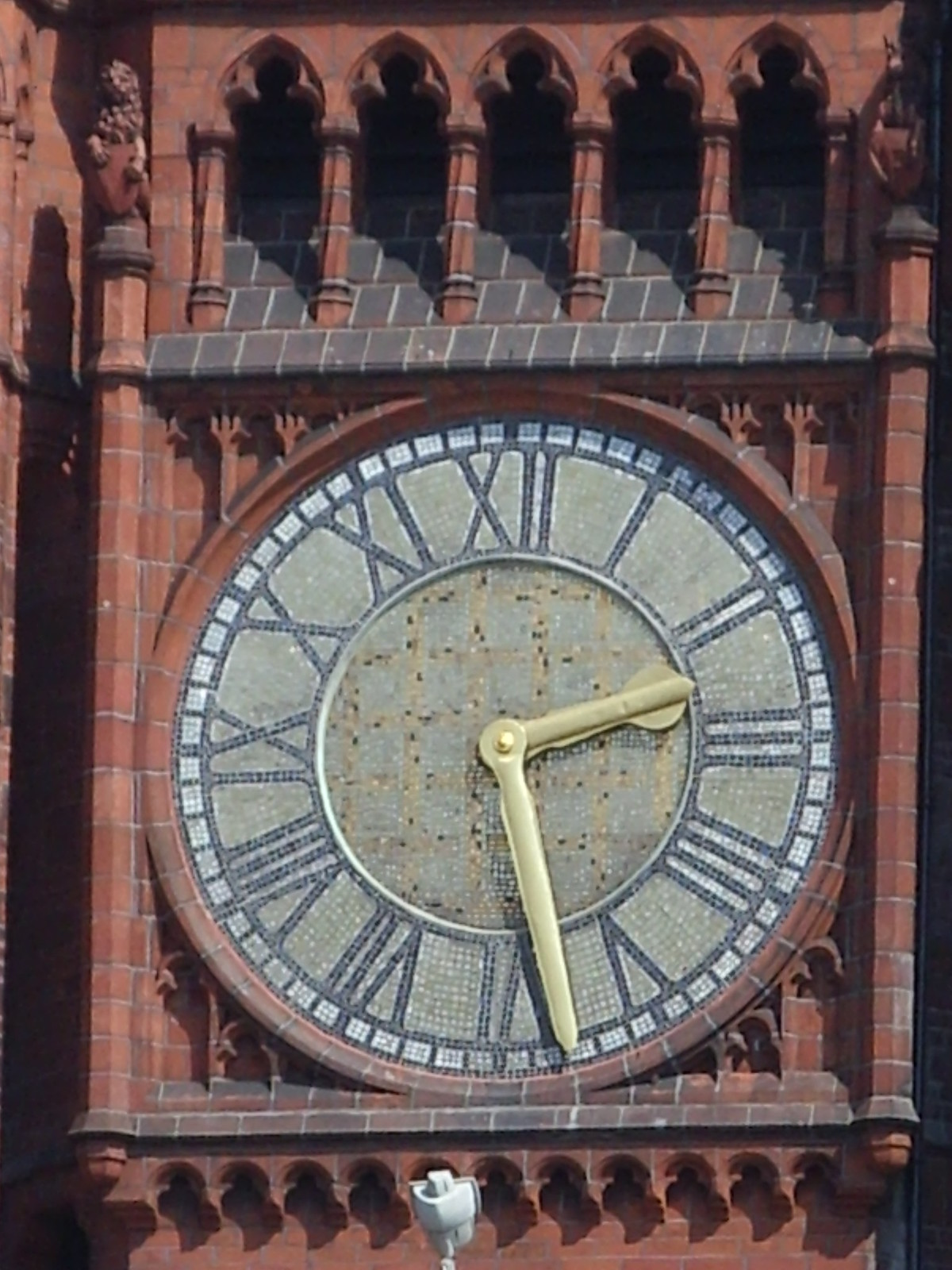This is a detailed photograph of a clock tower on a grand, European-style brick building. The building features elaborate architectural flourishes, including five arches at the top, with brick columns in between, made of brownish brick with a reddish hue. Above the clock, there are representations of knaves flanked by small stone lions. 

The clock face itself is large and gray, encircled by small white squares. The numbers are Roman numerals, styled like a mosaic in blue tiles. The clock's hands, made of brass and colored in yellowish gold, show the time as approximately 2:29, with the hour hand pointing between 2 and 3 and the minute hand between 5 and 6. The entire composition captures a mixture of historical elegance and intricate details.